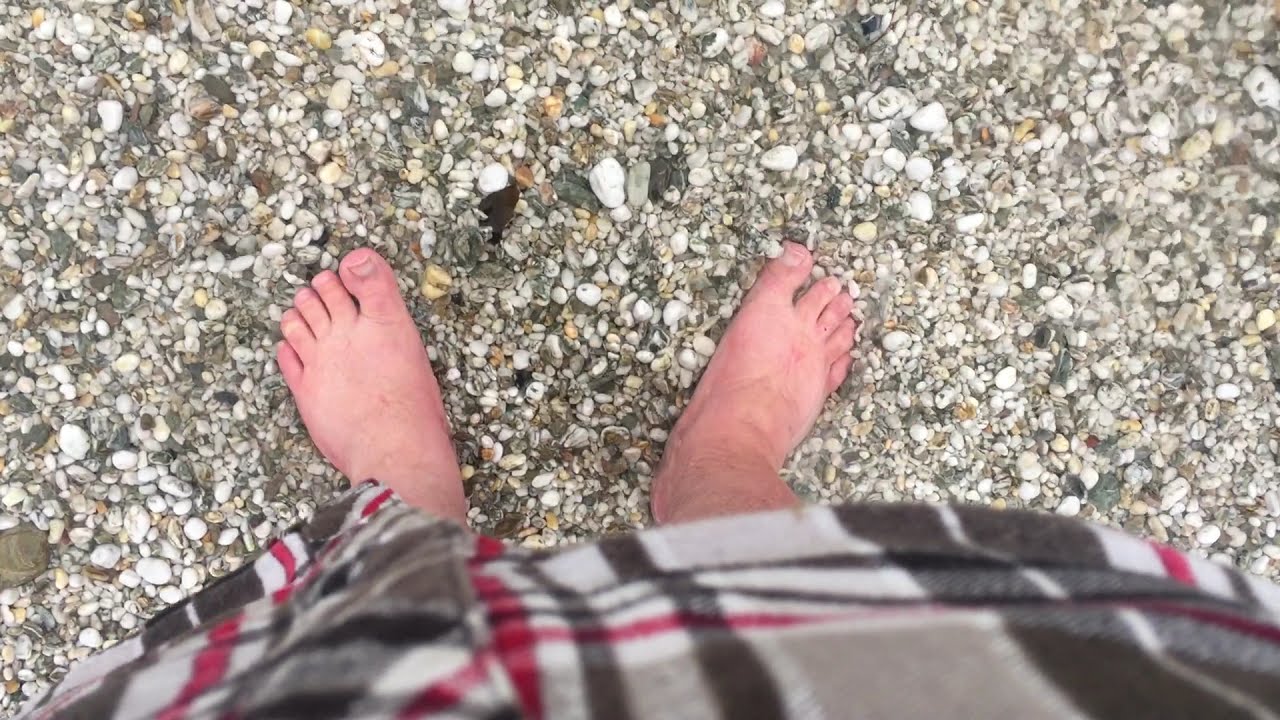The image captures a top-down view of an individual's bare feet, with toes splayed outward and each foot pointing slightly in opposite directions—the right foot bent more to the right. The person is standing on a surface composed of variously sized, multi-colored pebbles and cobblestones, including some larger stones and broken seashells, creating a textured and visually diverse flooring. The surrounding ground features darker stones in the upper right-hand corner. The person is wearing a garment with a checkered and striped pattern that extends below the knees, possibly resembling pajama bottoms or a long striped shirt. The garment includes black, white, red, and gray colors, and has long vertical black bars interspersed with thin red stripes and a mixture of gray, suggesting it is a heavy material suited for warmth. The intricate design of the garment and the bare feet set against the detailed pebble flooring create a rich, visually striking composition.